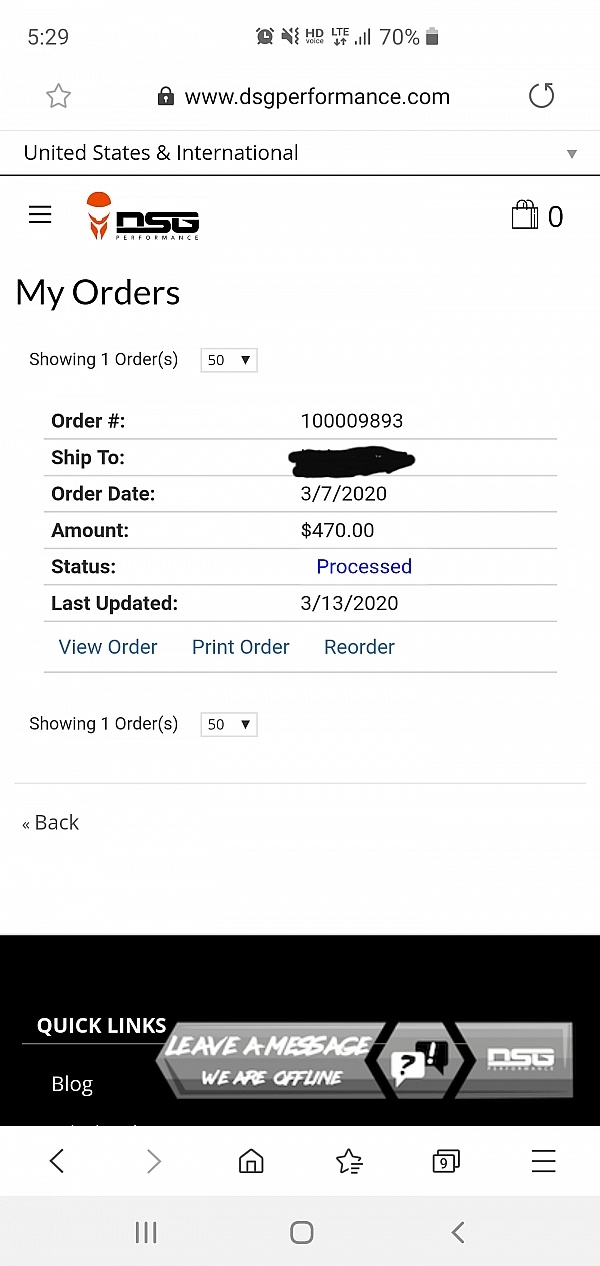A close-up view of a cell phone screen displaying a webpage from DSGPerformance.com. At 5:29 PM, with the device in silent mode and the battery at 70%, the screen shows various elements neatly arranged. On the left side is a star icon, while the site's logo, featuring red and black colors, is prominently displayed above three stacked lines for a pull-out menu. The central part of the screen features the site's name, "DSGPerformance.com," flanked by a refresh button on the right. Below this are links for "United States and International" shipping options with a drop-down menu.

On the top-right corner, there's a shopping basket icon with a zero next to it, followed by the text "My Orders," indicating one order. The order summary shows order number 100009893, dated March 7, 2020, with an amount of $470 and a status of "processed" updated on March 13, 2020. Personal details under "Ship to" have been redacted. Below this, options to view, print, or reorder are presented in teal blue buttons.

A black banner runs along the bottom of the screen, and a back link is located on the left side, just above the banner.